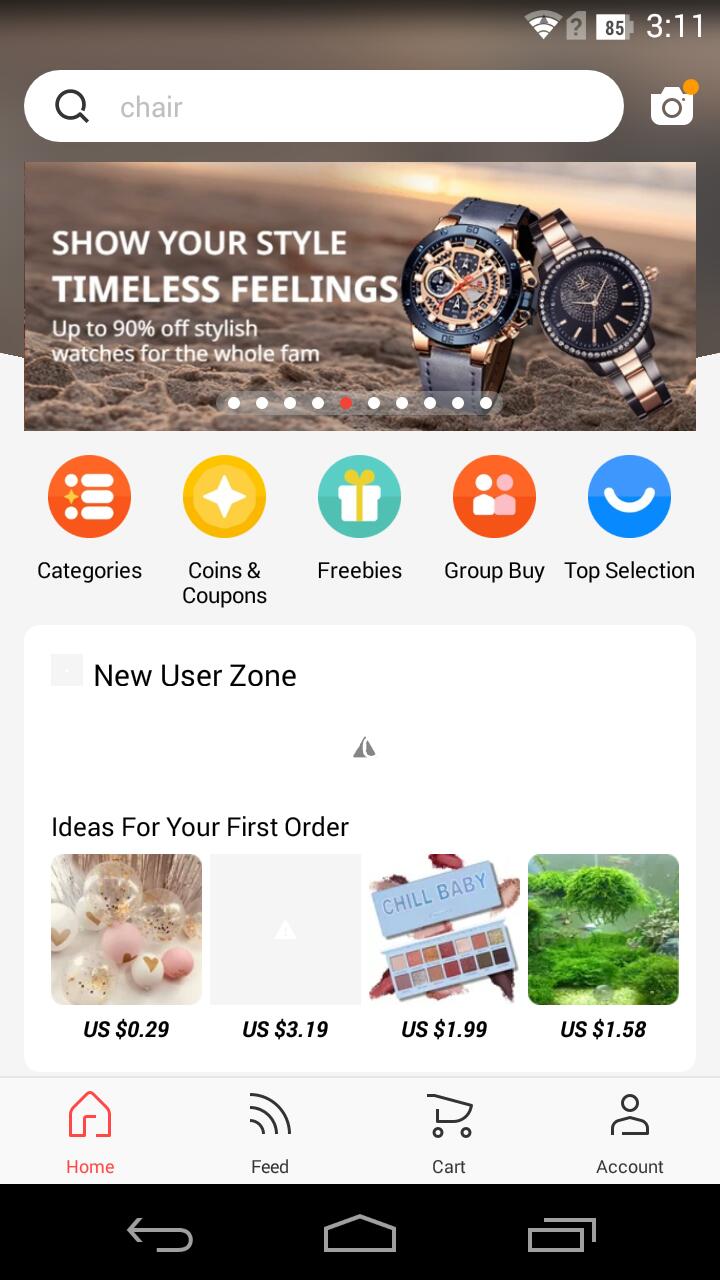This screenshot reveals a view of an e-commerce app interface taken at 3:11 PM, when the device battery stands at 85% and is connected to a moderately strong Wi-Fi network. The app, which specializes in a wide variety of products including watches, freebies, group buys, makeup, and balloons, targets users with personalized suggestions. 

Prominently featured at the top of the screen is an ad encouraging the user to "Show your style, timeless feelings," showcasing two elegant watches—one men's and one women's—both in black with gold embellishments. 

Below the ad, five main navigation categories are displayed: 
1. Categories
2. Coins and Coupons
3. Freebies
4. Group Buy
5. Top Selection

A "New User Zone" section follows, suggesting introductory offers for first-time buyers with prices listed at $0.29, $3.19, $1.99, and $1.58, indicating this user has not yet made a purchase via the app.